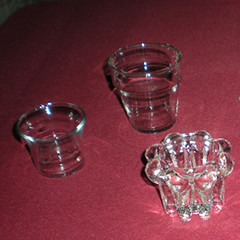This image features a close-up of three distinct glass objects placed on a red background, likely a red tablecloth. The objects include two plain glasses and one decorative glass. The first plain glass, located to the left, has a simple, straight design similar to traditional barware or shot glasses. The second plain glass, slightly larger and positioned towards the center-right, shares a similar straightforward style. The third glass, situated at the bottom right and most brightly lit, is highly decorative with scalloped edges and intricate segments, resembling a crown. Its reflective crystal design makes it difficult to discern its exact shape. The overall lighting highlights the glass details and casts a light image around their bases, enhancing the intricate design of the most ornate glass. All three glasses appear to be empty, and the photograph's quality suffers slightly from reflections, making some features a bit hard to see.